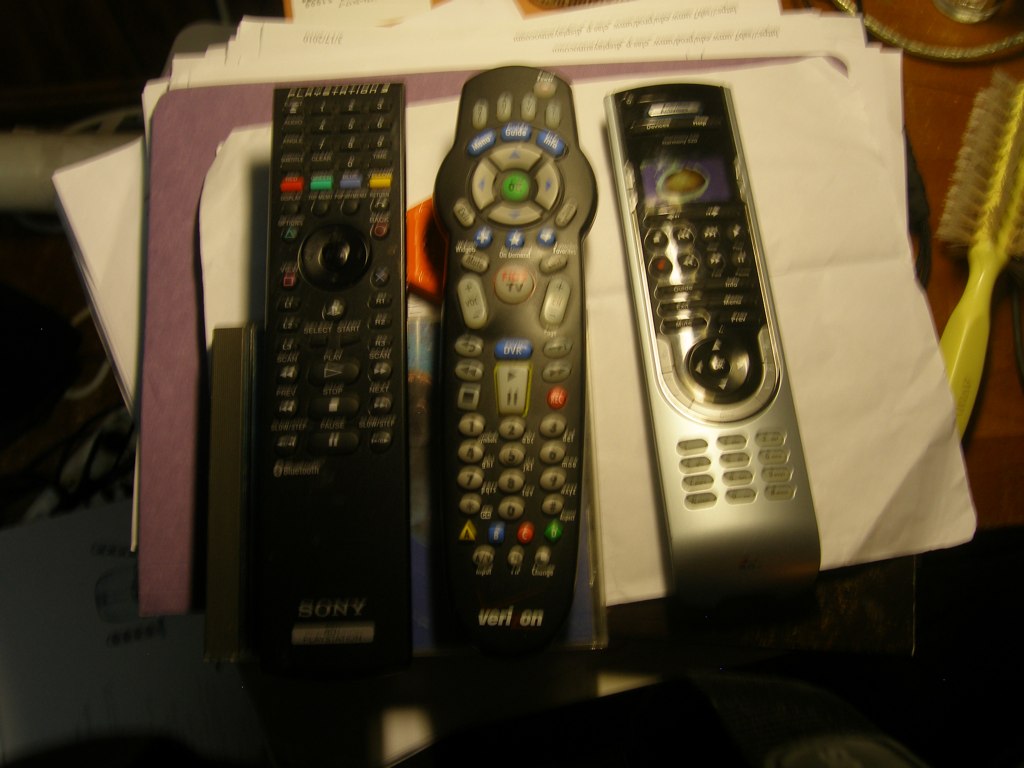The image depicts three distinctly colored remote controls arranged on top of a stack of papers, which sit on a purple folder filled with various documents. On the far right, there is a yellow hairbrush with gray bristles. To the edge, you can spot a brown hat with gold embroidery resting on a dark wooden table. The leftmost remote, marked "Sony," features a number pad, multicolored buttons in red, green, blue, and yellow for various functions, and standard playback controls. The central remote, labeled "Verizon," also has a numeric keypad and playback buttons, including a row of color-coded buttons: yellow, blue, red, and green. The remote on the right is silver and black, equipped with a small LCD screen at the top and a variety of buttons, indicating it could be for multiple devices. Despite the blur and lack of focus, the photograph clearly captures these details in an indoor setting.